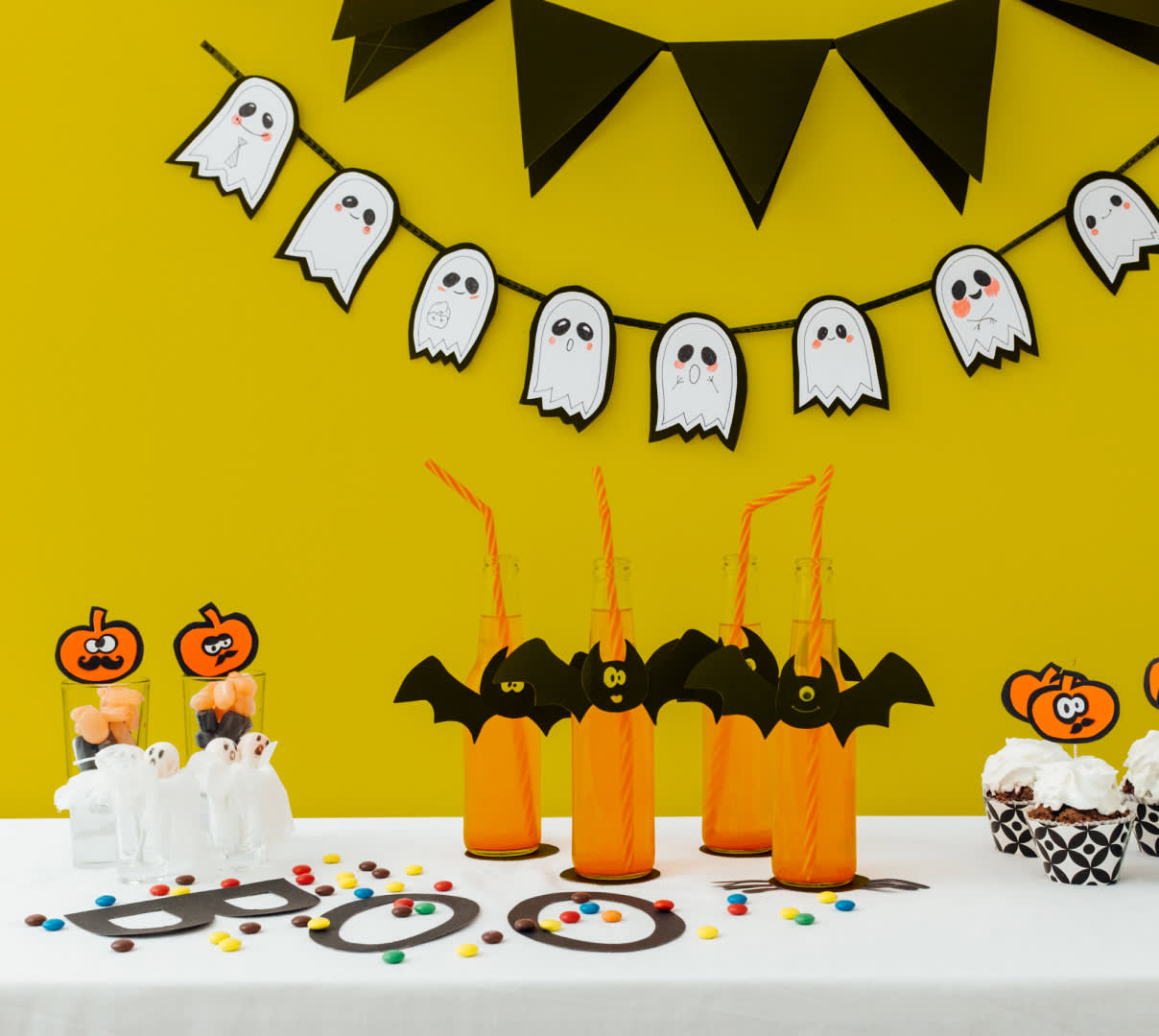This detailed image captures the festive setup of a Halloween party table set against a solid yellow wall adorned with a string of playful, white ghosts that resemble Pac-Man ghosts, complete with varying expressions like smiles and tears. Above the ghosts, a series of triangular black banners hang like a festive choker. The rectangular table at the bottom is covered with a pristine white tablecloth and is scattered with colorful M&M's.

On the left side of the table, there are glasses filled with black and orange candies, each topped with whimsical pumpkin figures sporting mustaches and bug eyes. The word “Boo,” crafted from large letters, spans the table amidst the candies but is slightly tilted downward, with the O's designed to resemble eyes.

In the center of the table, behind the "Boo," are tall soda bottles filled with orange liquid, each decorated with a smiling bat face and fitted with a bent orange licorice straw. To the right, short sundae cups with cream-filled chocolate bases are topped with whipped cream and little pumpkin toothpick signs, encased in black and white diamond-patterned holders with black dots.

Additional details include the presence of ghost-themed marshmallow treats sprinkled around the table, enhancing the overall spooky yet playful Halloween atmosphere.